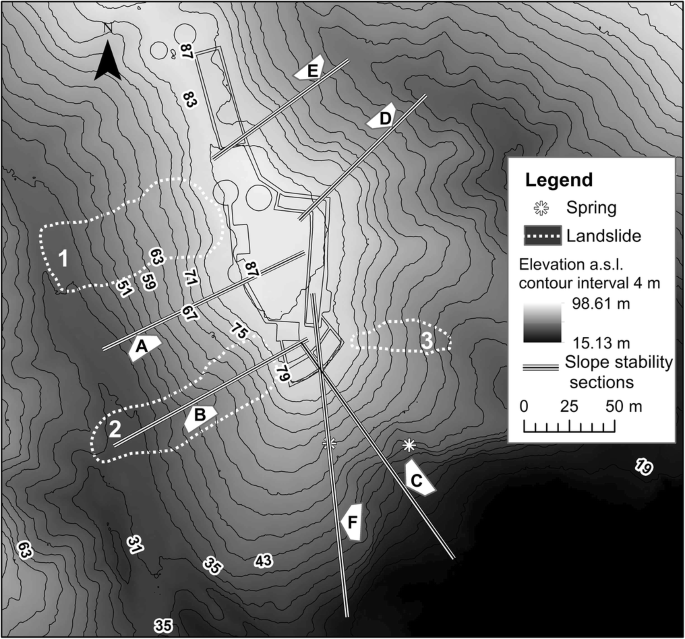This black-and-white topographical map provides a detailed view of an elevated landscape, characterized by contour lines indicating various elevation levels. Centered around a shape resembling a guitar, the terrain stretches from the upper left to the middle of the image, with contour lines rippling outward. To the map's right is a white square containing the legend. The legend includes symbols: an artwork of a snowflake labeled "spring," a dotted line signifying "landslide," and different shades of gray to indicate elevation changes—the darker the color, the lower the elevation, and the lighter the color, the higher the elevation. The legend also provides specific measurements:
- Elevations: 15.13m, 98.6m, 4m contour interval
- Slope stability sections

A horizontal ruler at the bottom of the legend measures distances from 0 to 50 meters, with the midpoint marked at 25. The map’s background is primarily white with varying gray shades, and it is marked with numbers and alphabetical letters to indicate specific points of interest. The bottom right of the map features a black area, contrasting with the rest of the light tones.